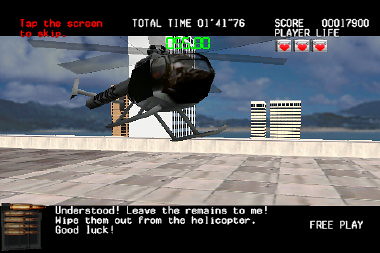This image is a horizontal, rectangular, color screenshot from an older-style, pixelated video game. Central to the frame is a black helicopter with gray propellers, seemingly poised to land or take off from a gray-blocked helipad on a building's roof. The scene is set high above a cityscape, with tall skyscrapers towering in the background and a distant coastline featuring the sea, a beach, and low hills, suggesting an elevated perspective.

The game's user interface is prominently displayed, noticeable by its somewhat fuzzy, pixelated graphics. At the top of the screen, a black bar spans around a fifth of the frame, containing various details: in the upper left-hand corner, red text reads "Tap to skip," while white text in the center shows "Total time: 01'49"76." To the right, the score is prominently displayed as "000017900." Below the score, there's a label "Player life" followed by three boxes each containing a heart icon.

Additional text is visible both above and below the game scene. A black bar at the bottom contains white dialogue text stating, "Understood! Leave the remains to me. Wipe them out from the helicopter. Good luck." In the lower right corner of the screen, the words "Free play" are displayed in white, emphasizing the game's free play mode. The overall composition gives off a nostalgic vibe, amplified by the pixelated texture and retro UI elements, set against an engaging aerial action scene.